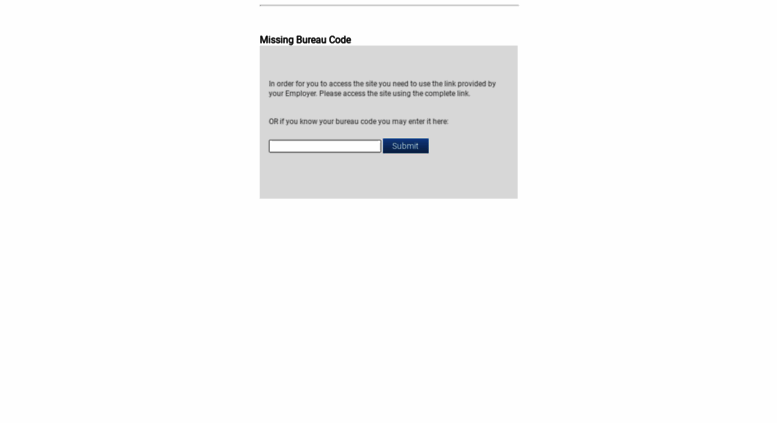The image is a small, structured informational graphic. At the top, there is a thicker gray line, followed by a white background. In bold black font with capitalized initial letters, it reads "Missing Bureau Code." Below this text, there is a large gray box containing instructions in smaller, grayish-black font. The instructions state: "In order to access the site, you need to use the link provided by your Employer." 

Following this, there is another directive: "Please access the site using the computer link." This is followed by approximately two lines of blank space. Below this, in capital letters, is the word "OR," followed by the text: "If you know your bureau code, you may enter it here." Adjacent to this text box is a field where users can enter their bureau code. Directly beside this field, there is a rectangular, dark blue button with thin white font that reads "Submit," with the 'S' capitalized. 

The largest font on the image is "Missing Bureau Code," which appears to be in bold and approximately size 16. All other text is around size 12.